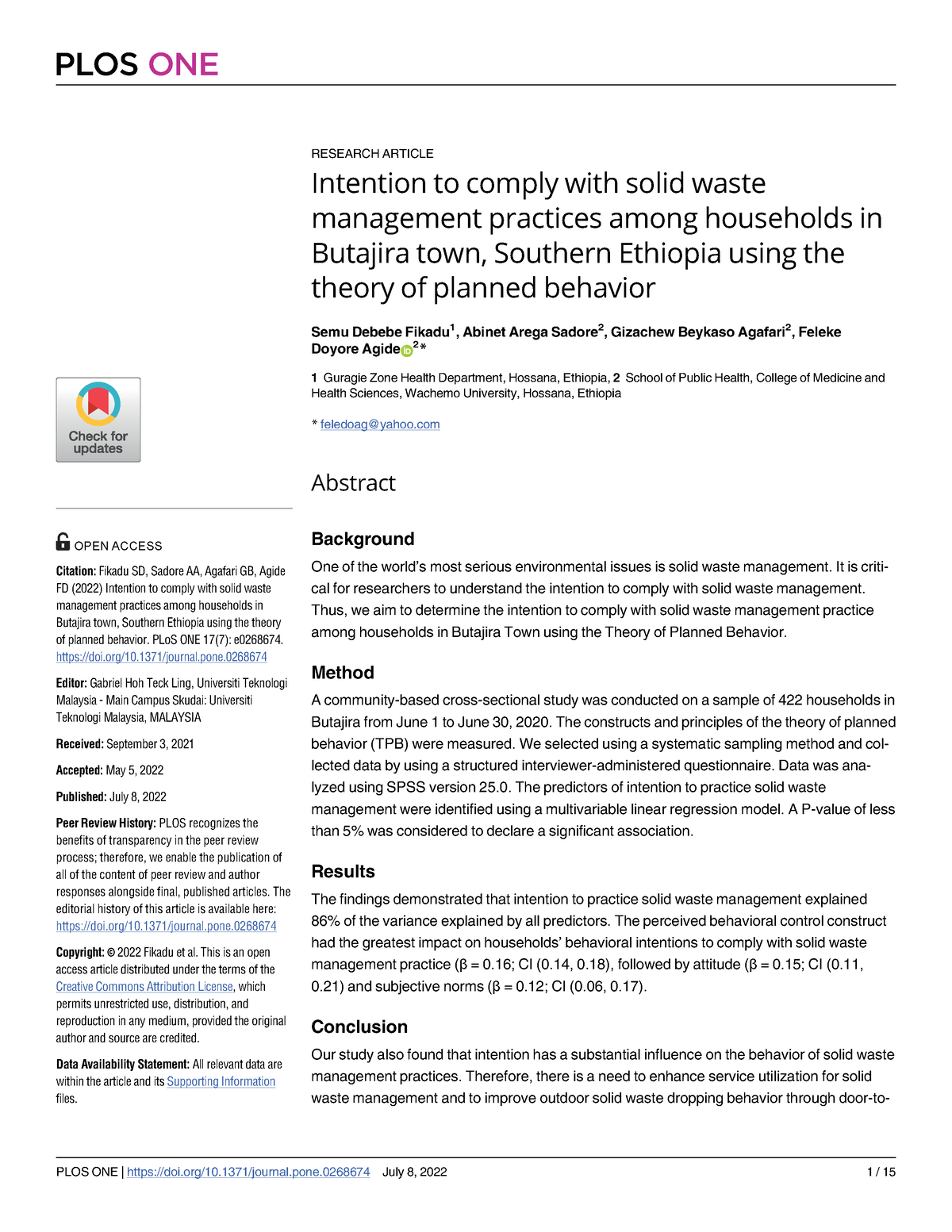The image depicts a webpage from the journal PLOS ONE. At the top of the page, "PLOS" is prominently displayed in dark gray letters, while the "ONE" is written in bold, capitalized pink letters. Below this header, the article title reads, "Intention to Comply with Solid Waste Management Practices Among Households in Butajira Town, Southern Ethiopia: Using the Theory of Planned Behavior."

The content of the article is organized into sections including the background, methods, results, and conclusion. However, the text in these sections appears quite small and is difficult to read in the image.

On the left side of the page is a clickable symbol designed for updates. This symbol features a circle that is half greenish-blue and half yellow. Inside this circle, there appears to be a red-colored badge or insignia.

At the bottom of the webpage, there is a section with blue letters, contrasting with the predominantly dark gray text used throughout most of the page.